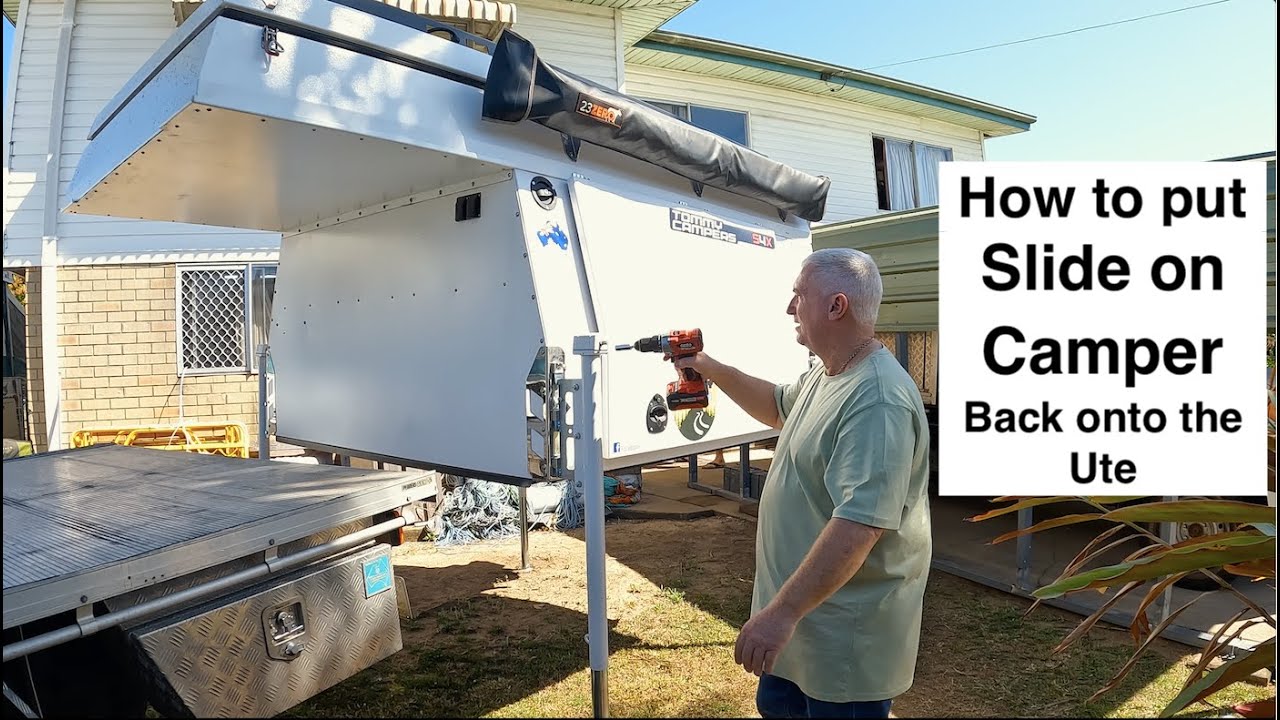The image depicts an older, somewhat plump man with short white hair, wearing an untucked, light mint green shirt and blue jeans. He is standing outdoors on a lawn, surrounded by green grass and brown soil patches, bathed in daylight. The man is holding an orange handheld drill and appears to be working on a white camper shell that is propped up on stilts, separate from a truck with a flatbed metal back. A white square with black text overlays the right side of the photo, stating "how to put a slide on camper back onto the ute." In the background, there is a two-story house with white upper walls and lower walls featuring brown brick patterns, including various windows with both glass and sliding designs. The scene is framed against a clear blue sky, emphasizing the sunny outdoor setting.